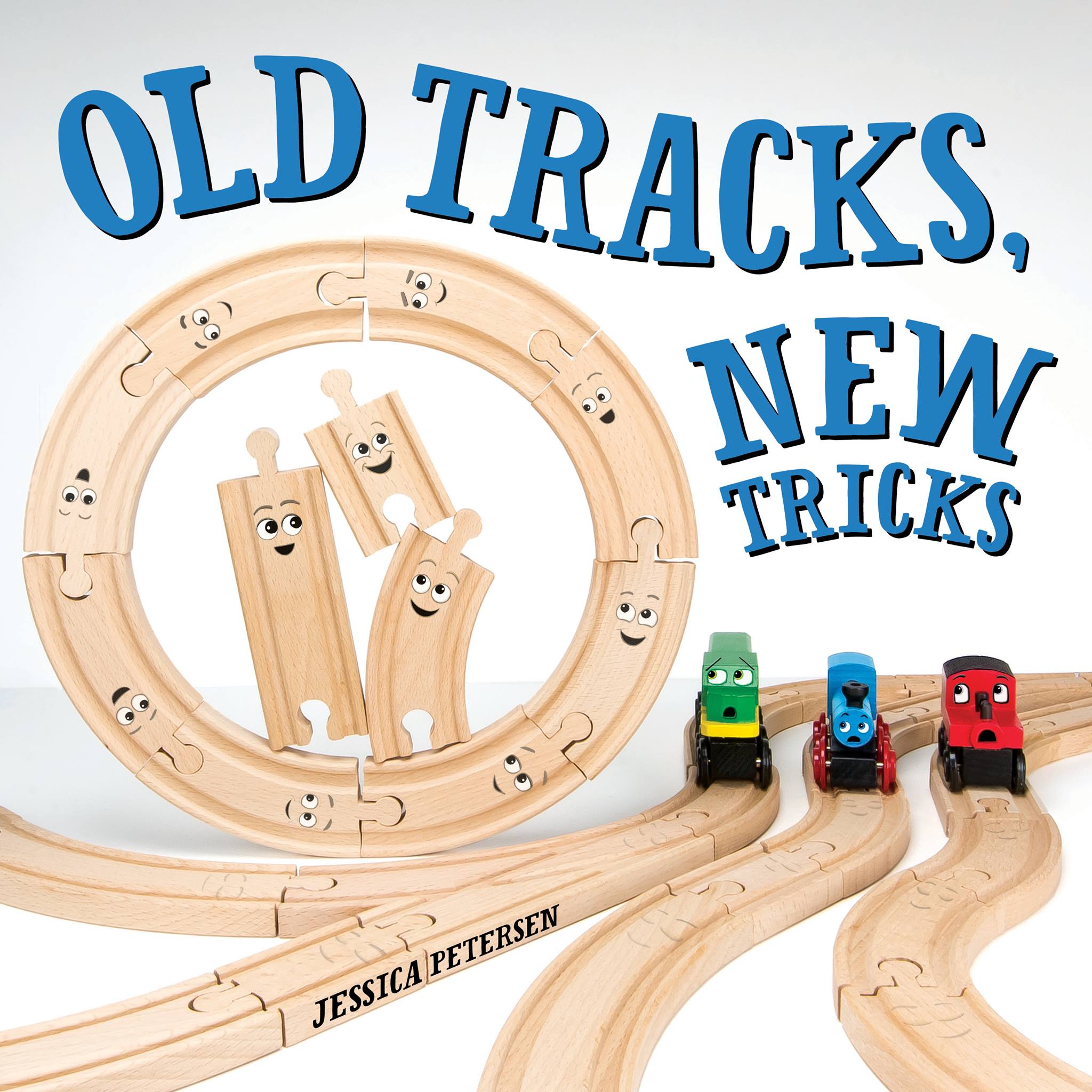The image is the cover of a book titled "Old Tracks, New Tricks" by Jessica Peterson, featuring Thomas the Tank Engine. Thomas the Tank Engine, along with a red train and a green train, are each on separate tracks. The green train's track has an interesting fork ahead, suggesting multiple possible routes. Additionally, on the left side of the cover, pieces of track are arranged in a circle, each adorned with a cheerful smiling face. In the center of this circle, three other track pieces also have smiling faces. The text "Old Tracks, New Tricks" is displayed in dark blue, while Jessica Peterson's name is written in bold black text. The overall scene is portrayed in a joyful and inviting manner that would appeal to children. The image seems to combine elements of a storybook and a playset, highlighting the playful and creative potential of the wooden tracks.